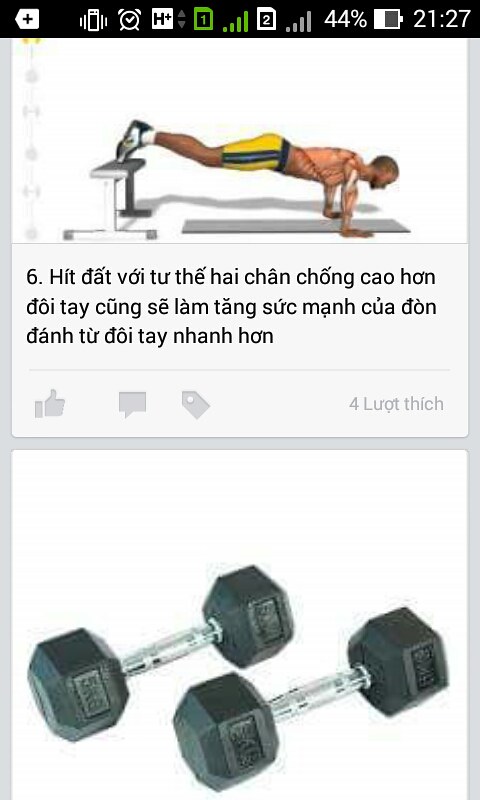This is a detailed two-part image, captured as a screenshot from a smartphone, as indicated by the icons showing 44% battery life and other emblems at the top. The upper half of the image features a diagram of a man performing elevated push-ups with his feet on a bench. The man, depicted in profile, is wearing yellow shorts with a dark stripe and sneakers. His upper body is shown with an anatomical view displaying muscles and bones, accompanied by Vietnamese text beneath it and marked with the number six. The man has dark brown, short crew-cut hair and is shirtless. In the lower half of the image, there are two horizontal dumbbells, each featuring silver handles and black weights on both ends. The text and imagery suggest detailed anatomical study and exercise instruction, emphasizing the precision and focus on both the push-up form and dumbbell weights.